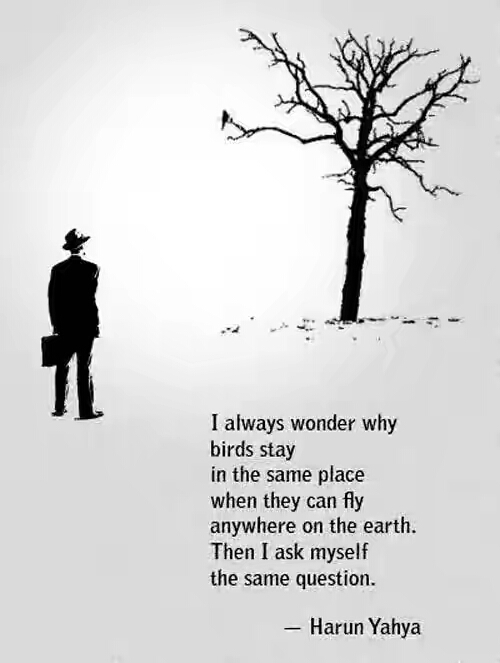The image depicts a minimalist black and white stencil drawing set against an off-white background. In the top right section, a solitary, leafless tree stands starkly, resembling a somber Halloween tree. A small bird perches on one of its branches. On the left side of the image, a man dressed in a formal black suit, carrying a briefcase, and wearing a hat, stands gazing up at the tree, as if pondering deep thoughts. In the bottom right corner, the quote in black text reads: "I always wonder why birds stay in the same place when they can fly anywhere on the earth. Then I ask myself the same question." It is attributed to Harun Yahya. The entire composition has a contemplative, motivational tone, typical of reflective posts often seen on social media platforms.